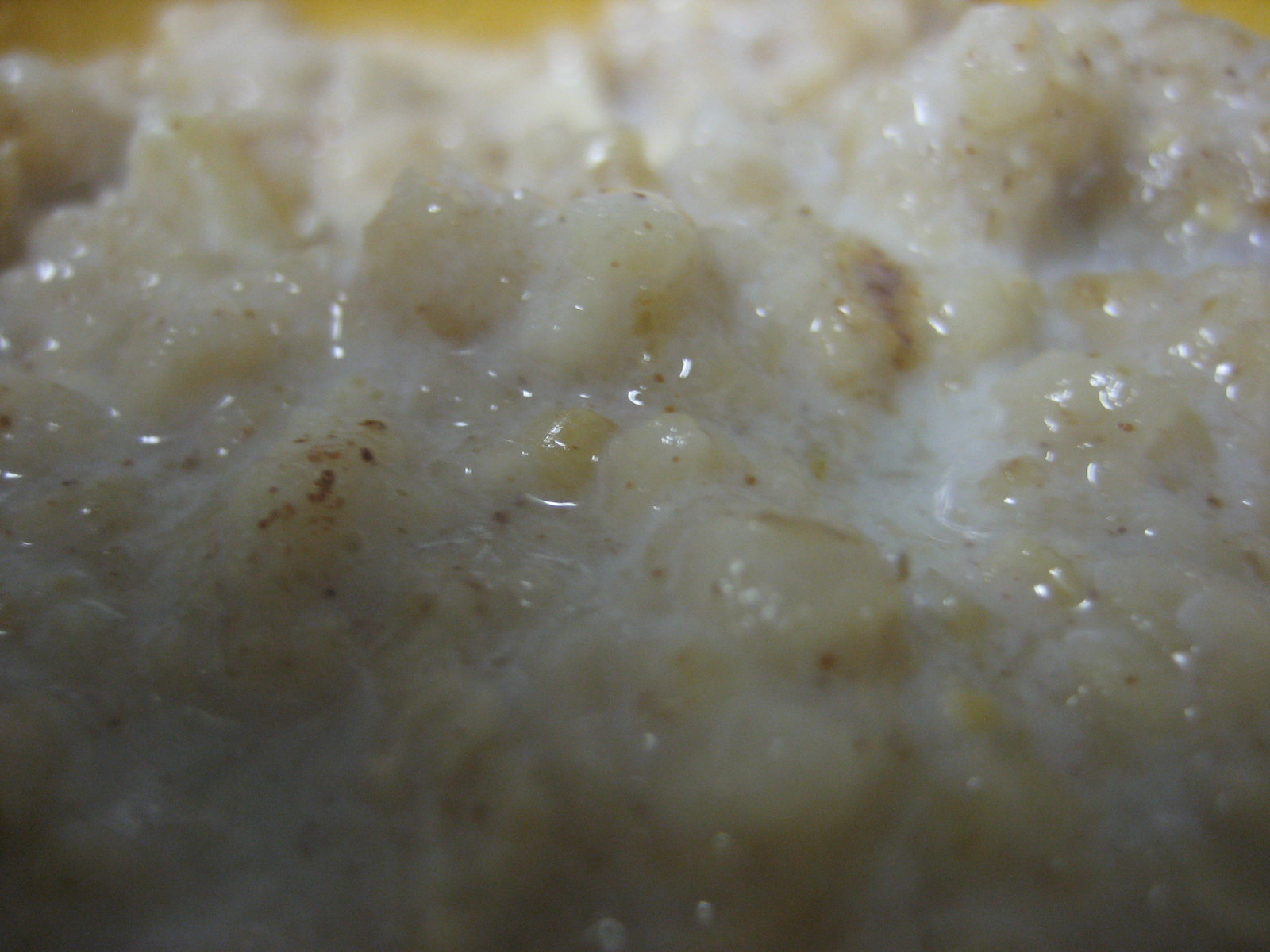The image is a close-up shot of a wet, lumpy, and creamy food that appears to be either oatmeal or cream of wheat. The dish has a light brown to yellowish hue, with a notably shiny and almost slimy appearance due to a liquid or sauce mixed throughout. Scattered across the surface are tiny, darker reddish-brown specks, likely cinnamon. The focal point of the image is centered, while the edges are blurred, drawing attention to the food's texture and color contrasts.